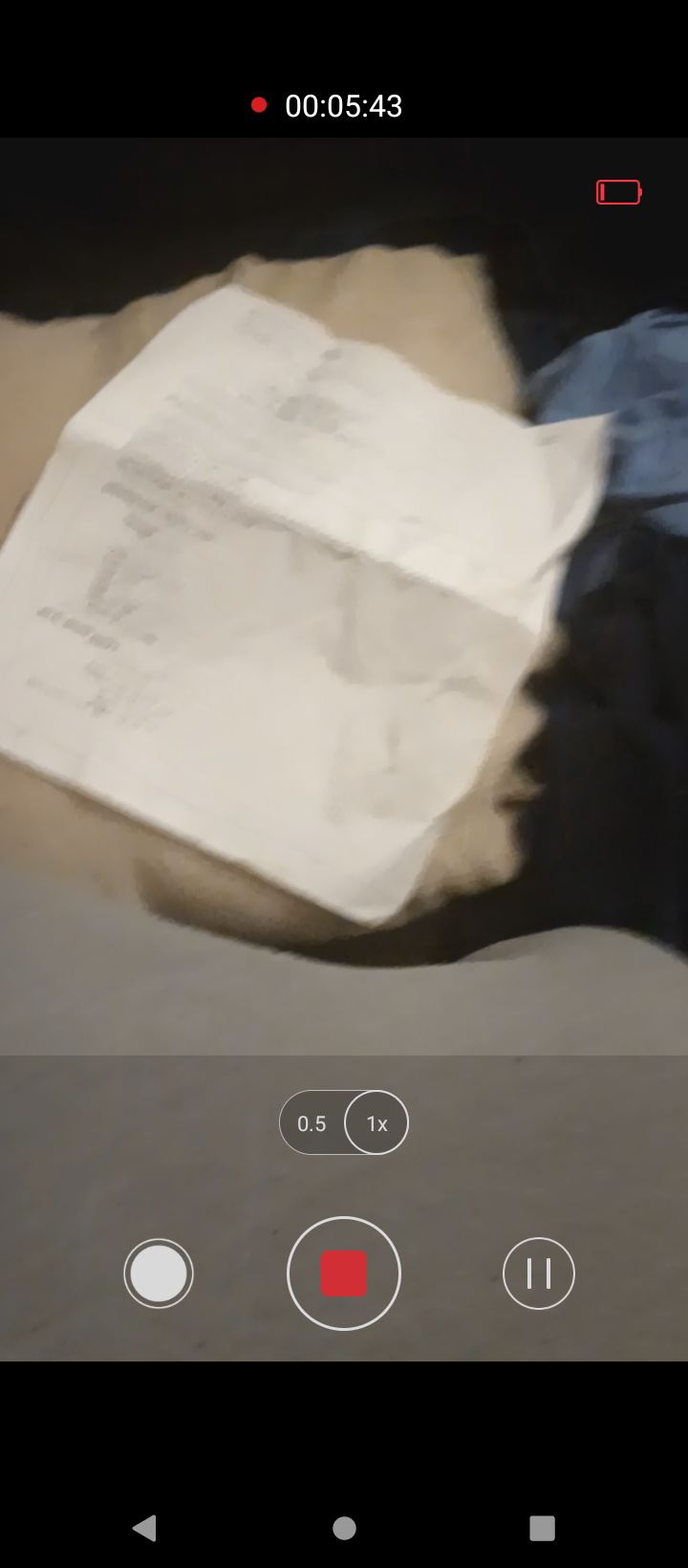The image appears to be a screenshot capturing a segment of a phone’s display while showing a blurry photograph. 

At the top, there is a black band featuring a red dot followed by a timestamp reading "00:05:43". This is likely an indication that a video is being recorded. To the right, there is a small red rectangle, possibly indicating a low battery or recording status.

The blurry photo in question seems to show several folded items of clothing. The topmost item appears to be tan pants. Next to it on the left is a partially visible light blue garment. On the right, a black piece of clothing is folded. Placed atop these clothing items is a piece of white computer paper. The paper, which has visible horizontal fold marks, is unfolded and slightly wrinkled. It appears to contain typed text that is illegible.

Below the image, there is a wider gray bar. Within this bar, on the left, there's a capsule-shaped button labeled "0.5" and a circle labeled "1x" in a darker shade of gray. Adjacent to this, on the right, are two white circles, one with gray elements inside, and a red square.

Towards the bottom, there's another black band featuring a gray triangle, a gray circle, and a gray square—these likely represent playback control icons.